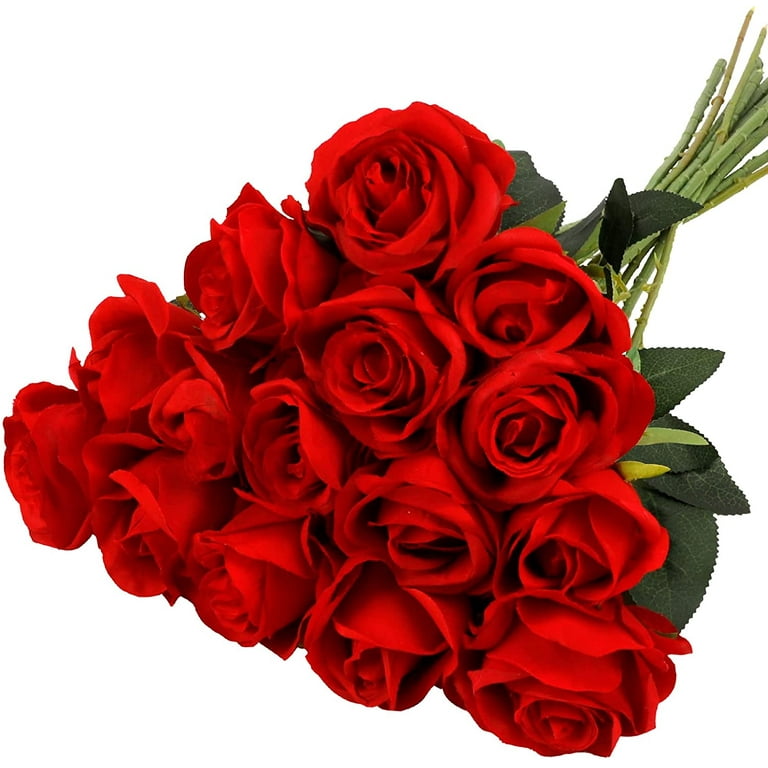A detailed photograph depicts a bouquet of 15 deep ruby red roses arranged in a pyramid-like or triangular formation against a white background. The flowers are viewed from above, showcasing their lush, multi-petaled heads all neatly bundled together. Each rose looks vibrant and healthy, with a crisp red hue that suggests they are freshly cut. The stems, pruned and free of thorns, extend toward the upper right corner of the image, displaying a light green color and small, dark green leaves that frame the bouquet. The roses are uniform in size, forming a symmetrical design: five roses on the bottom row, followed by another five slightly smaller roses above, then three roses, and finally a pair of roses at the top. The stems and leaves enhance the picture's aesthetic, but there is no additional text or lettering present. The overall impression is one of carefully arranged, glowing red roses, perfect for a visual celebration of their beauty.